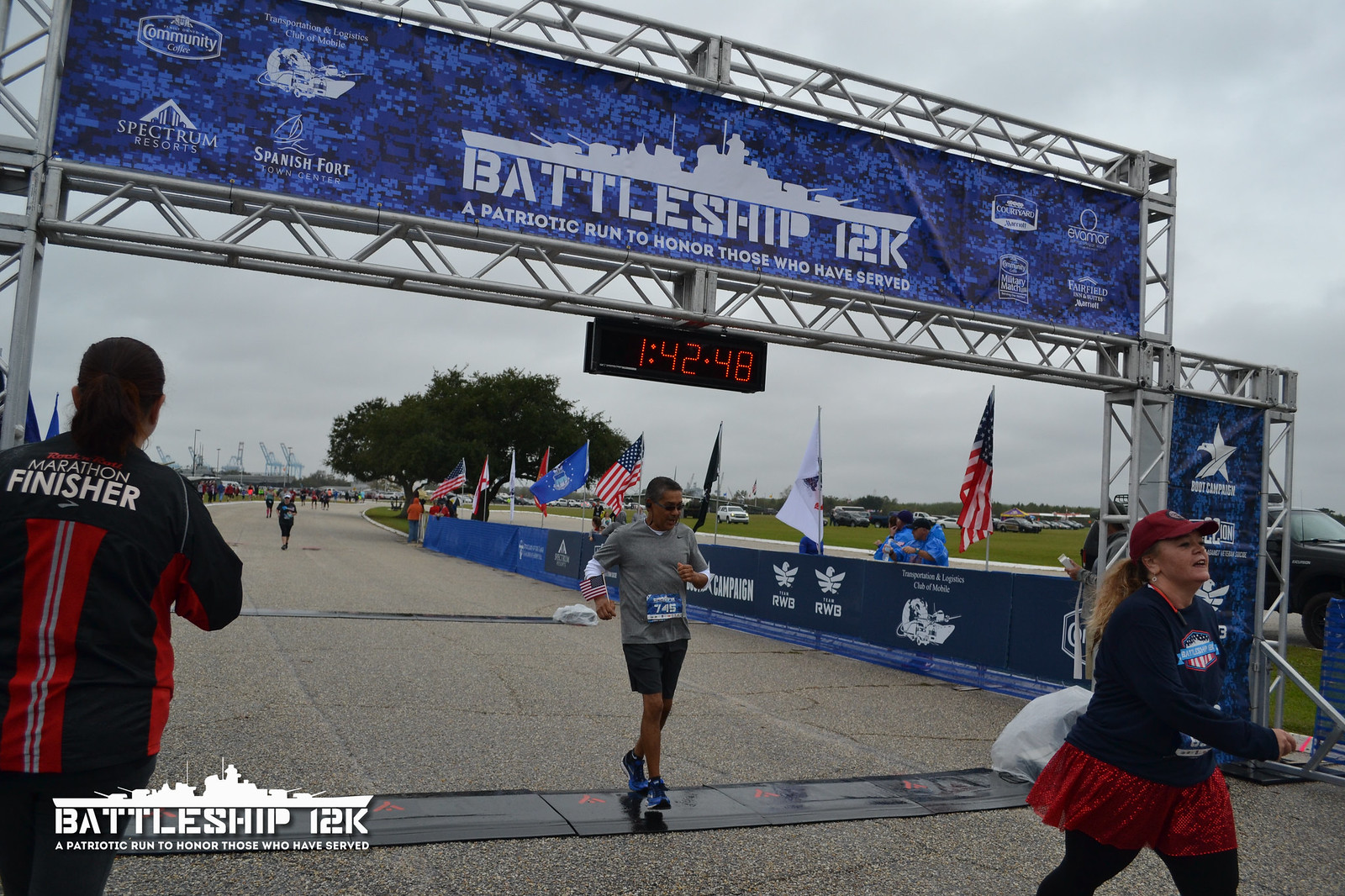The image captures the finish line of the Battleship 12K race, a patriotic event to honor those who have served. Central to the scene is a large blue banner emblazoned with a shadowed image of a battleship and the race's name. Below this banner, a digital clock displays the time of 1:42:48. In the forefront, a woman with long blonde hair, wearing a red hat, blue sweatshirt, red skirt, and black tights, has just crossed the finish line. Close behind her is an older gentleman dressed in a gray short-sleeved shirt over a white long-sleeved shirt and black shorts, carrying an American flag. Alongside the road, patriotic signs and banners featuring sponsor logos are prominently displayed. The race route is bordered by a blue-bannered gate, adorned with grass and flags, adding to the celebratory atmosphere. Off to the side, a person with their back to the camera wears a jacket that reads "Marathon Finisher," contributing to the overall spirited environment of the race.